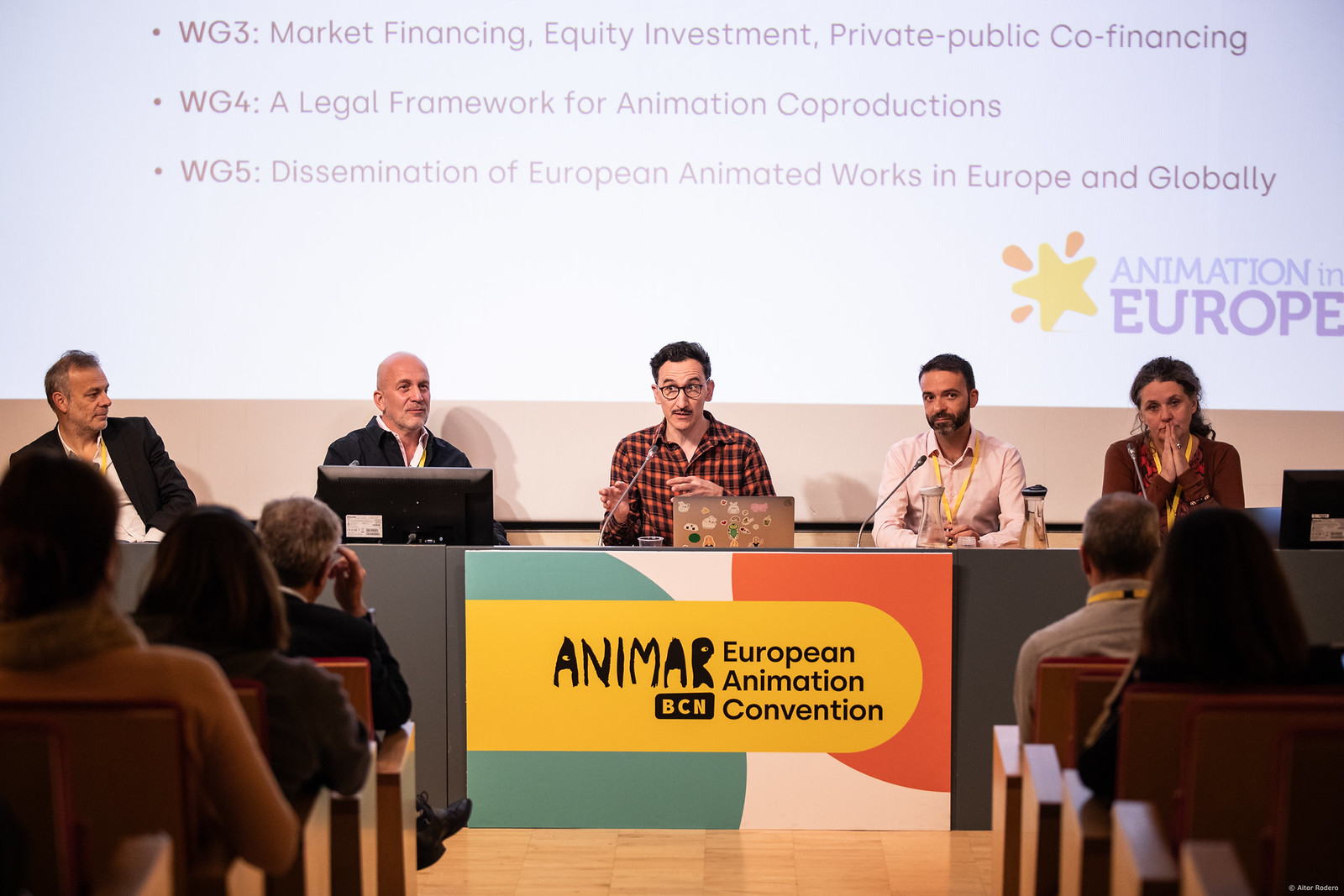A diverse panel of five people is seated behind a desk at the front of a room, facing an audience. The man on the far left, wearing a black jacket and white shirt, with gray hair, is looking to his right. Next to him sits a bald man, also in a black jacket, in front of a black screen. The middle person is wearing an orange and black plaid shirt, black glasses, and has his hands raised, appearing to speak into a microphone with a laptop adorned with stickers in front of him. To his right is a man in a peach-colored shirt with a yellow lanyard, sporting a full beard and short black hair, his hands resting on the desk. On the far right is a woman with brown hair pulled back, wearing an amber shirt with a yellow lanyard and clasping her hands in front of her face.

In front of the central speaker, a sign reads "NMR, European Animation Convention, BCN" with a colorful background in green, yellow, and orange hues. The polished wooden floor complements the wooden pew-like seats filled with audience members, enhancing the formal setting.

Behind the panel, a projector screen displays critical points of the presentation: WG3 – Market Financing, Equity Investment, Private-Public Co-Financing; WG4 – A Legal Framework for Animation Co-Productions; and WG5 – Dissemination of European Animated Works in Europe and Globally. The backdrop emphasizes the collaborative and international focus of the convention on animation in Europe.